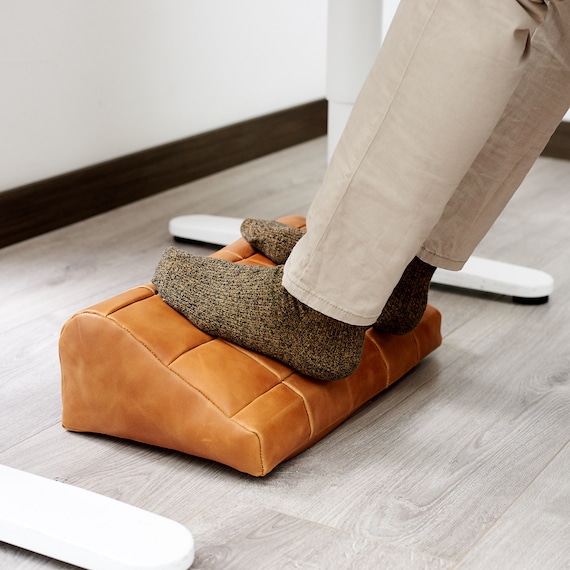This image is a product demonstration showcasing a foot wedge designed to be used under a desk. The wedge is made from a soft, light brown or tan leather with a quilted pattern. The photograph features a person seated at the desk, likely off image to the right, with their legs visible from the calves down. They are wearing khaki pants and woolen socks. The desk has white, inverted T-shaped legs and the setting includes light gray wood panel flooring with a white wall and dark brown molding in the background. The intentional setup and clear presentation suggest the photo is aimed at promoting the foot wedge, likely for an online product listing.